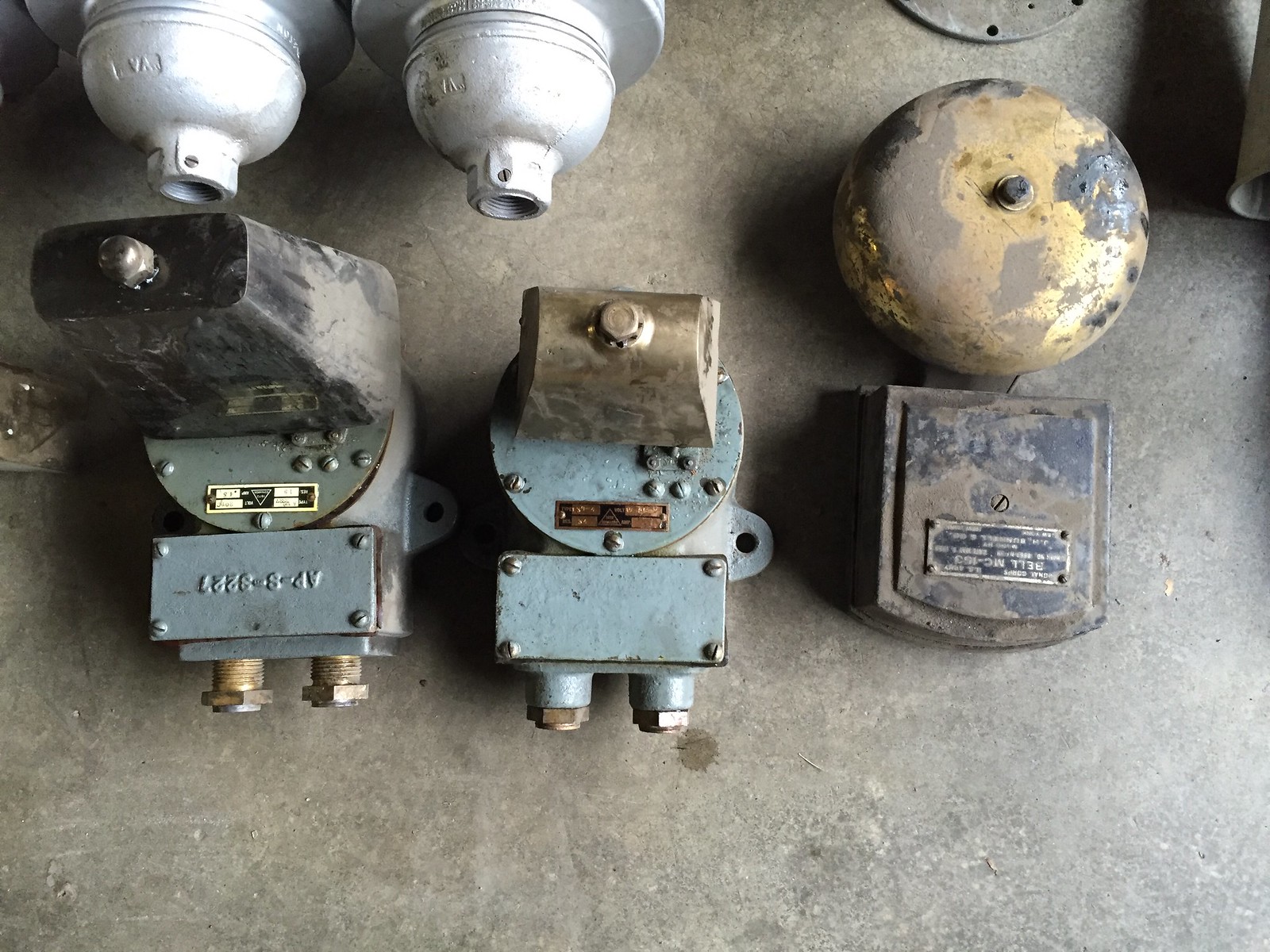This photograph showcases an assemblage of three distinct, vintage fire alarms set against a concrete surface. On the left, a large rectangular bell, weathered and tarnished with age, is mounted atop a mechanical device featuring two sturdy brackets. Adjacent to it in the center, a slightly smaller yet similarly shaped rectangular bell rests on another bracketed mechanism. This bell shares the same antiquated, uncleaned appearance as its larger companion. Completing the trio on the right is a traditional, circular school bell, also considerably old and attached to a mechanical device. Each of these bells, be it the large rectangular, the smaller rectangular, or the round school variety, is connected to its respective mechanical mechanism designed for automatic ringing. The bells exhibit hues of brown, black, and blue, accentuating their vintage charm and historical utility.